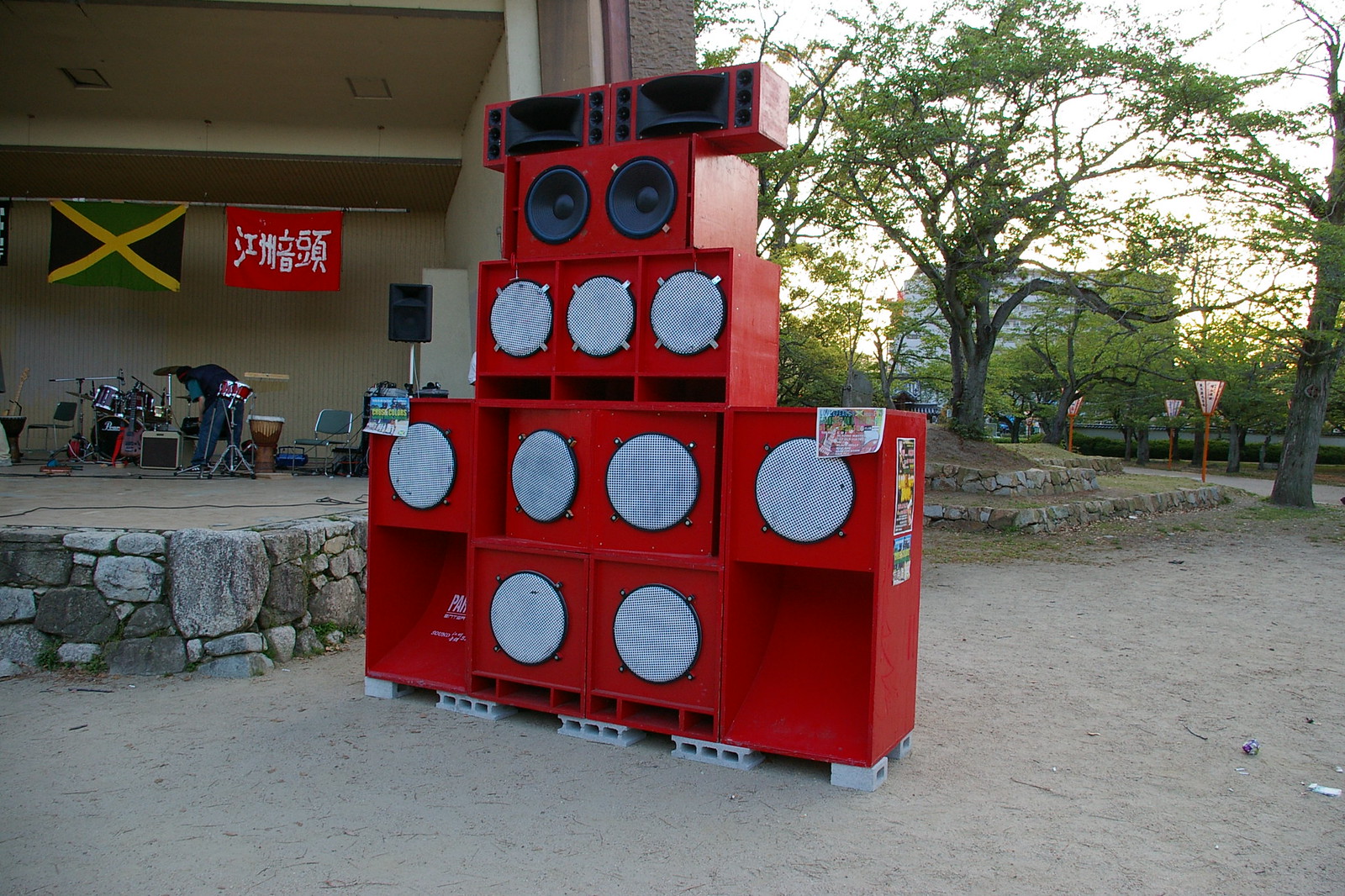In this outdoor photograph, captured under evening light, a strikingly tall and bright red shelving unit stands center stage. This shelf is composed of multiple rectangular compartments, each housing bright red speakers fitted with white mesh covers, all of which rest securely on flat cinder blocks. Higher up, a smaller wooden shelf with three compartments also contains these red speakers. Above this, an even smaller red shelf features black speakers, and at the very top, slightly wider shelves with flat rectangular black speakers complete the pyramid-like structure.

To the left, a platform edged with various sizes of rocks supports a stage. On the stage, a drum set is being inspected by a bent-over figure, and a collection of instruments — including an acoustic guitar and an electric guitar — can be seen, along with a black chair. Hanging above the stage are two flags: the Jamaican flag, featuring green, black, and yellow triangles, and a red banner with white Asian script.

The background features a park landscape with trees, a dirt path, and people walking near a building with street signs visible. The trees nearby have sparse leaves, and the sky, faintly illuminated, hints at the approaching dusk, adding a serene ambiance to the scene.